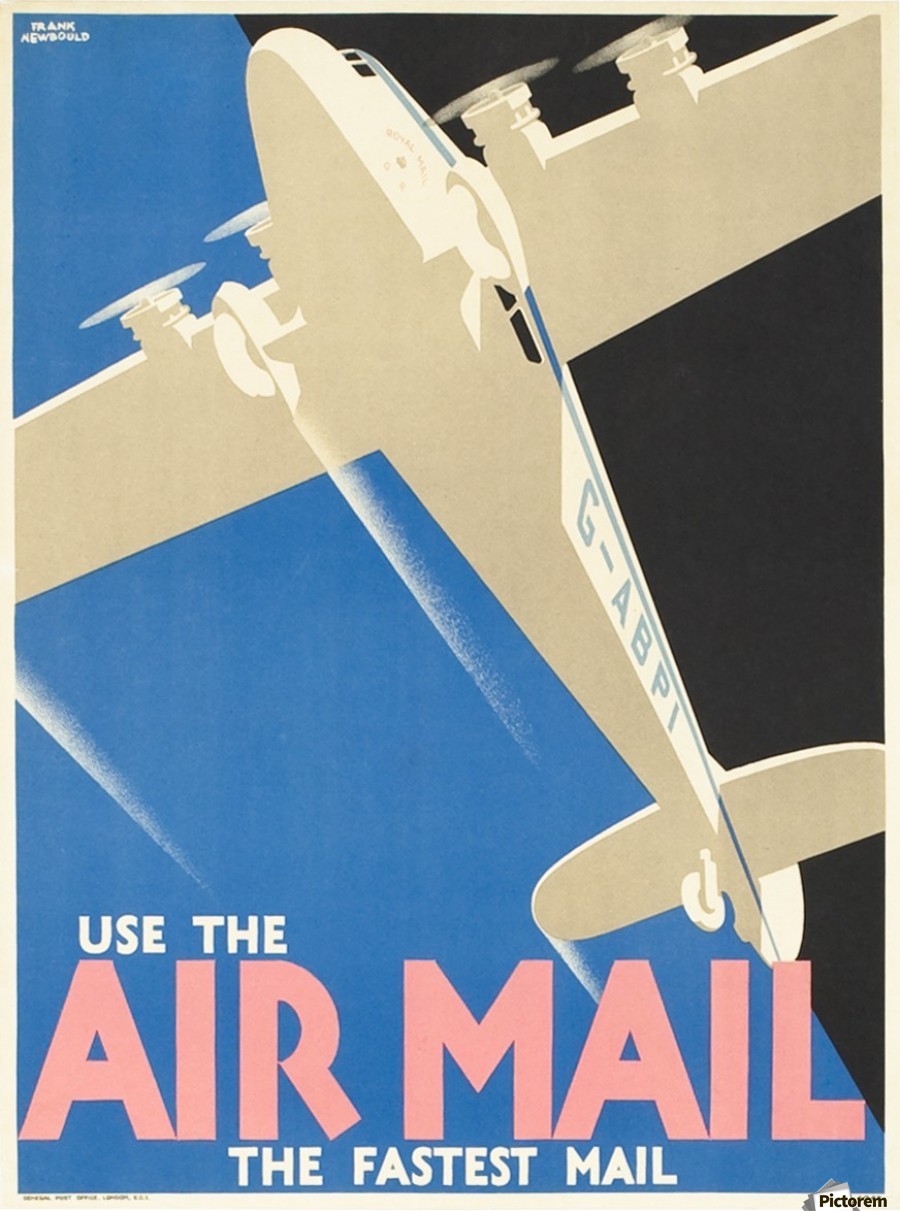The poster features a striking image of an airplane soaring diagonally upwards to the left against a backdrop split into a lighter blue sky on the left and a dark blue to black sky on the right, possibly symbolizing day and night. The rectangular poster is framed by a light brown stripe along the inside edges. The plane, primarily white with a light blue stripe down its side, bears the registration "G-ABPI" in blue text. It has black windows for the cockpit and side, and showcases four propellers, two on each wing set. Visible below the aircraft is bold text that reads "USE THE AIRMAIL" in pink, followed by "the fastest mail" in white. At the bottom right corner, the word "PICTORIUM" appears in black. Notably, the dividing line between the blue and black sections runs through the center of the image, emphasizing the airplane’s prominence as it moves across the contrasting skies.